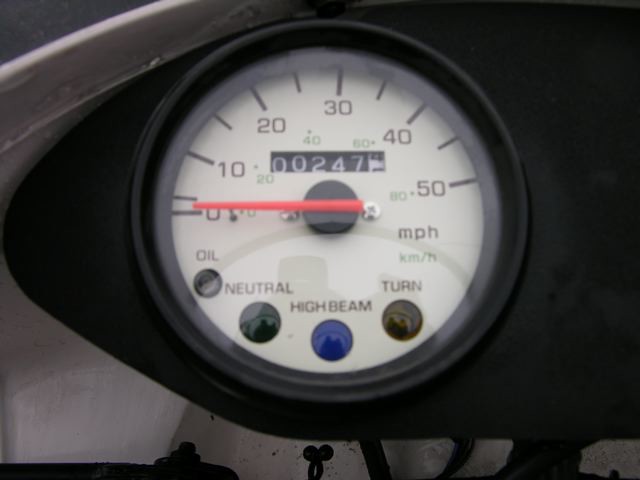This landscape-style image captures a close-up of a speedometer designed for a vehicle. The speedometer’s dial ranges from 0 to 50 miles per hour, marked in increments of 10. Each increment is highlighted with large black rectangles extending down from the dial's perimeter. A prominent red needle, long and slender, points towards the numbers, while the background of the speedometer is a crisp white. 

At the bottom of the dial, a small gray circle contains the word "OIL" in black font. To the right of it, a slightly larger green circle reads "NEUTRAL." Continuing rightward, there’s a blue circle labeled "HIGH BEAM," followed by a yellow circle indicating "TURN." 

Centrally positioned on the speedometer is a black rectangle, displaying the numbers "00247" in white font. This indicates the vehicle's total mileage or trip information. Surrounding the speedometer is a sleek black background, complemented by a silver shield-like dome covering part of the left side of the image, adding a metallic gleam to the overall composition.